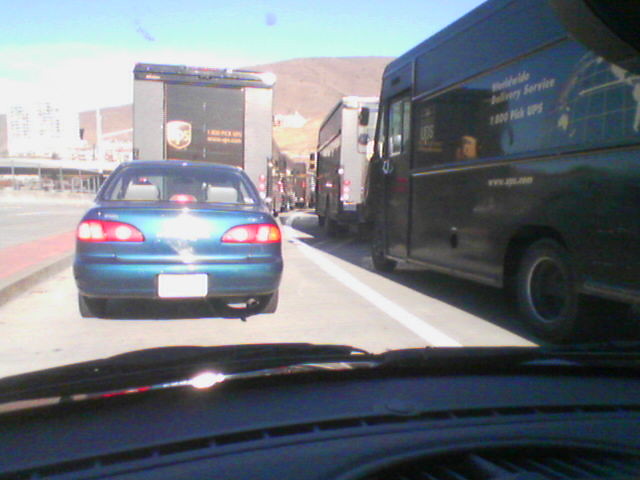This photo, taken from inside a vehicle in traffic, presents a busy, sunny day with a clear blue sky. From the driver's point of view, you can see the car's dashboard and windshield wipers at the bottom of the image. Directly ahead in the foreground, the hood of the car is partially visible. The main subject in front of the vehicle is an older, shiny blue sedan that resembles a Toyota Corolla. Its back end has a large glare, obscuring the license plate. Flanking the sedan is an array of UPS trucks; to its immediate right is one UPS truck, and ahead, the lanes are filled with a line of these brown delivery vehicles. The traffic seems dense, and to the right of the scene is a red median. In the background, beyond the cars, are light poles, buildings, a glimpse of a freeway, and a towering brown mountain under the bright, cloudless sky.